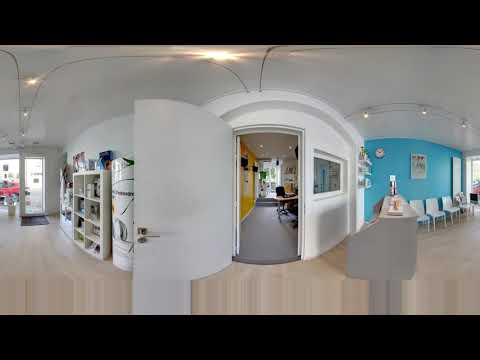The image depicts a panoramic view of what appears to be a waiting area or a retail-type space. The setting is predominantly white, with white walls and ceiling that create a clean, sterile atmosphere. The floor is a beige wood paneling, adding a touch of warmth to the space. On the far left, there is a door and a window that reveal a red car parked outside. Next to this, a white bookshelf laden with various items lines the wall.

Progressing from left to right, the focal point of the scene is an open door that leads into a room characterized by yellow walls, a chair, and a desk, suggesting it might be an office space. This office also features grey carpeting and darker wood paneling, contrasting the lighter tones of the waiting area. Above the office door, there is a window providing a view into this smaller space.

To the right of the office entryway, the wall turns blue and serves as a backdrop for several white chairs arranged in what seems to be a waiting area. A clock is mounted on this blue wall, adding a functional element to the scene. A piece of white artwork is also present, enhancing the aesthetic appeal. Towards the far right, another window partially obstructs the outside view, aligning with the spatial organization.

Overall, the panoramic nature of the image introduces some distortion, particularly visible along the lower portion. This comprehensive visual encapsulates the multifaceted space, merging the elements of a waiting area, an office, and a retail environment into a cohesive description.